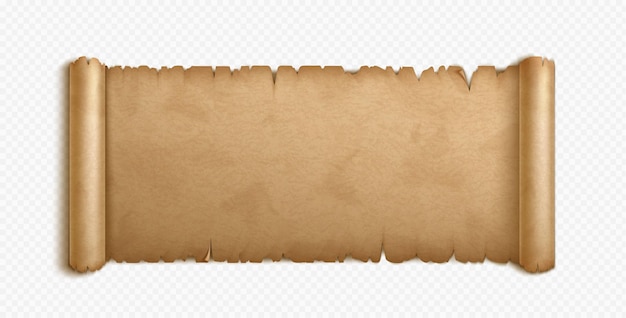This image depicts a computer-generated graphic of a medieval-style scroll, unrolled to display an empty parchment with frayed, jagged edges. The scroll, rendered in a light brown color, showcases its texture and shading, giving it a realistic appearance. Both ends of the scroll are rolled up, leaving the center portion visible and blank. The background features a gray and white diagonal checkerboard pattern, enhancing the digital and placeholder nature of the image. The lighting suggests a light source from the right, casting a shadow to the left. This scroll, likely intended for use in digital media such as games, websites, or graphic design projects, serves as a customizable element where users can add their own text or graphics.